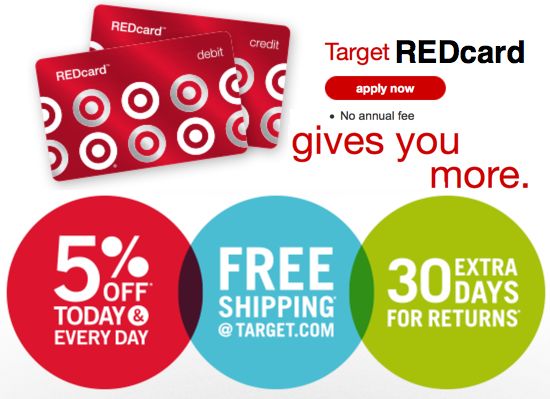This is an advertisement for Target prominently featuring their RedCard. At the top of the image are two solid red cards, one partially overlaying the other, each emblazoned with Target's iconic white circle and red bullseye logo. Accompanying the cards, the text "Target RedCard" is written in bold red, while "Red Card Debit" appears in black. 

A bright red circle containing the words "Apply Now" is also prominently displayed, emphasizing the ease of application. Beneath this, the ad highlights three main benefits of the RedCard, each within its own large colored circle. The first circle is red and states "5% off today and every day," overlapping slightly with the next. The second circle, in light blue, promises "free shipping at target.com." The third circle, in lime green, offers "30 extra days for returns."

The background of the advertisement is predominantly white, which enhances the visibility of the vivid red cards and text, making it unmistakably a Target promotion even without recognition of the logo.